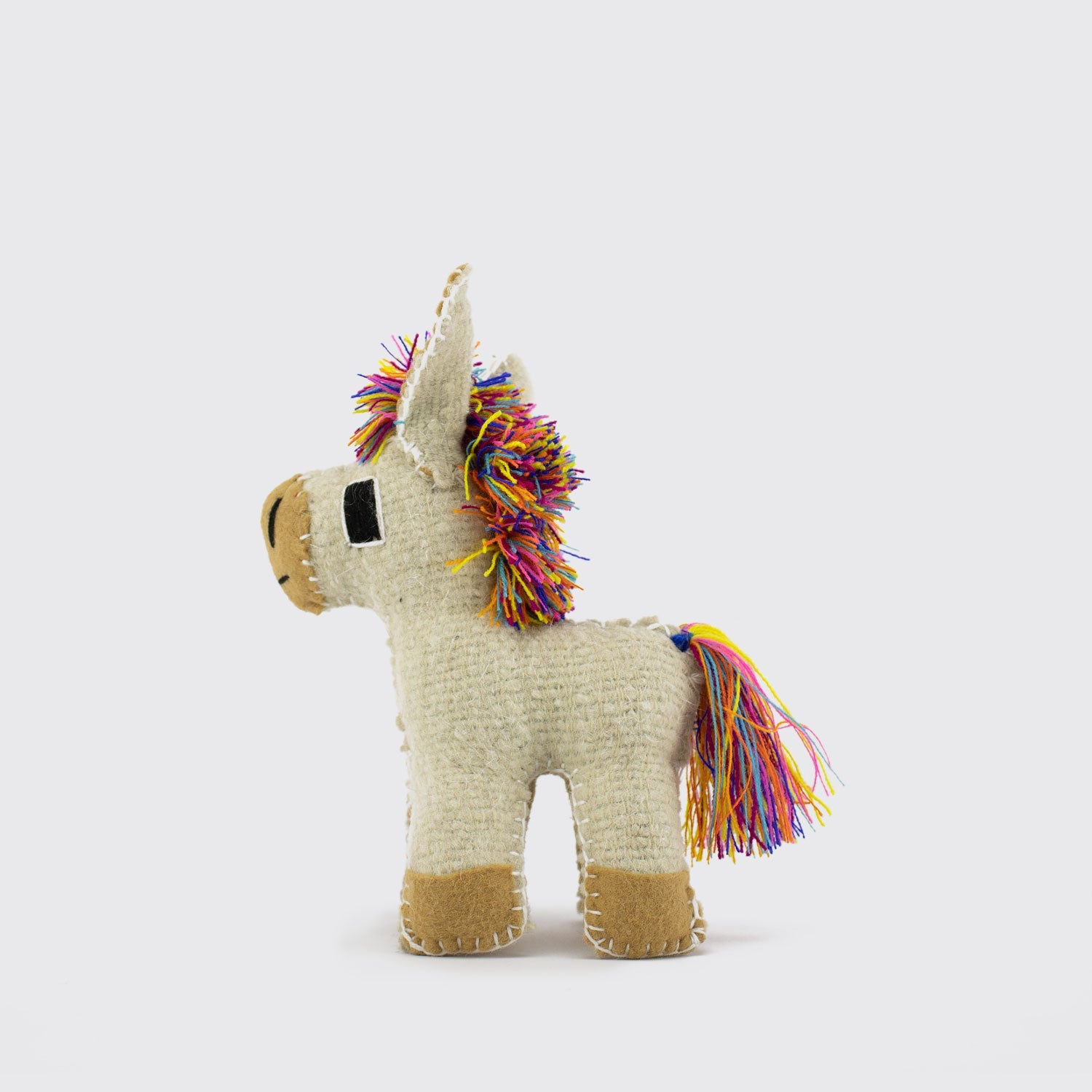The image depicts a handcrafted stuffed animal, likely a llama, characterized by its soft cream-colored body and detailed stitching. It has a distinctive face with a light brown felt-like nose stitched with white thread and adorned with black markings. Prominent features include rectangular black eyes with white borders and pointed ears. The llama’s light brown paws mirror the nose with similar white stitching. Its mane and tail are composed of vibrant, rainbow-colored threads including shades of yellow, orange, blue, pink, purple, and green. The background is a light blue, and the animal is photographed from a sideways angle, highlighting its wooly texture and detailed craftsmanship.